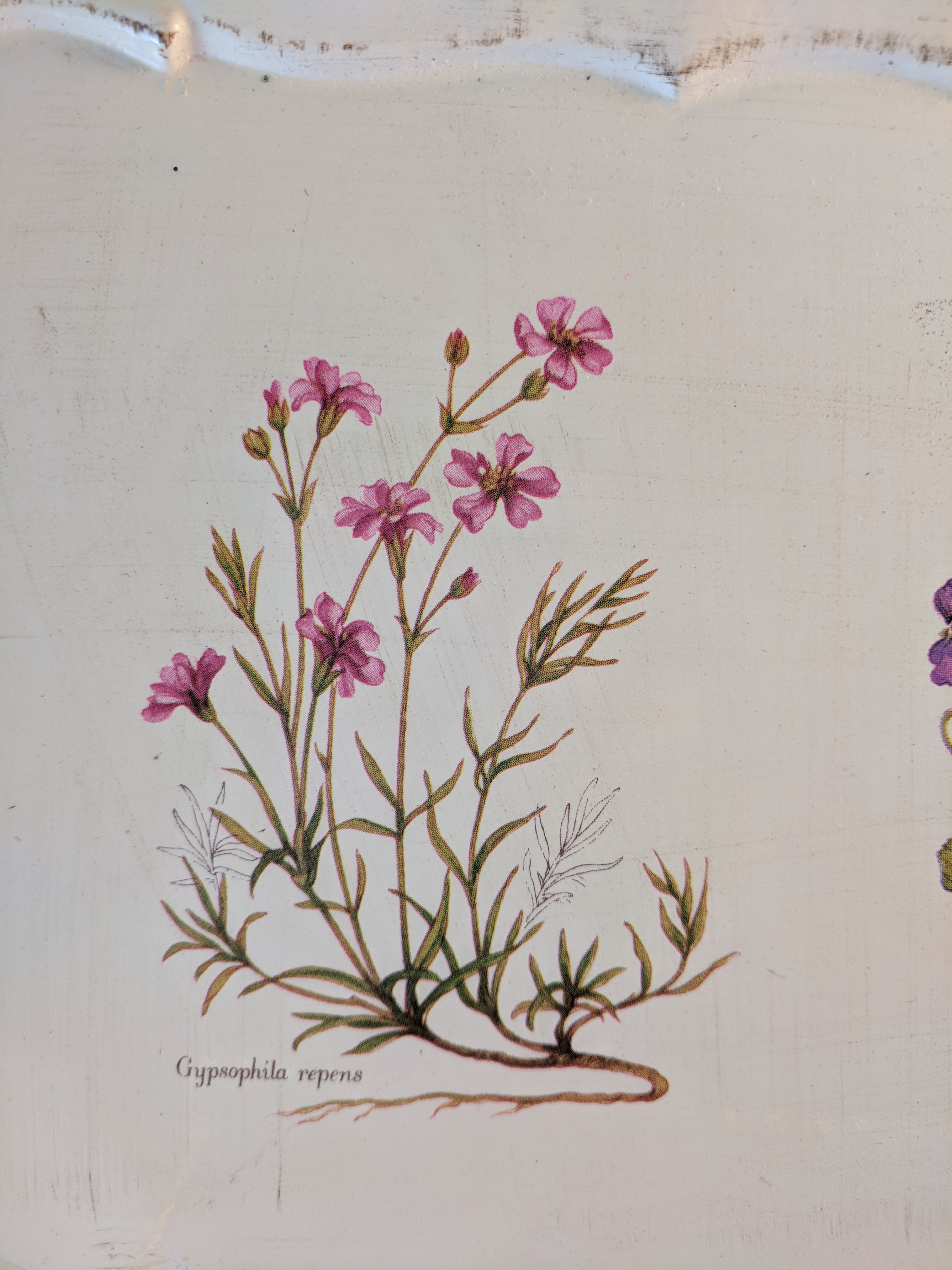This image appears to be an older illustration, possibly from a vintage botanical book, depicting a flowering plant identified as Gypsophila repens. Set against an off-white or beige background, the plant's intricate details are meticulously rendered. It features green leaves, some of which have a hand-drawn appearance with a tannish-green tint. The plant is adorned with blooming flowers that have pink petals and yellow centers, and also includes unbloomed buds. The roots, showing a tannish-brown color, are prominently displayed, curving downward. Additionally, on the right side of the illustration, another barely visible plant shows its purple flowers and some leaves, hinting at its presence.